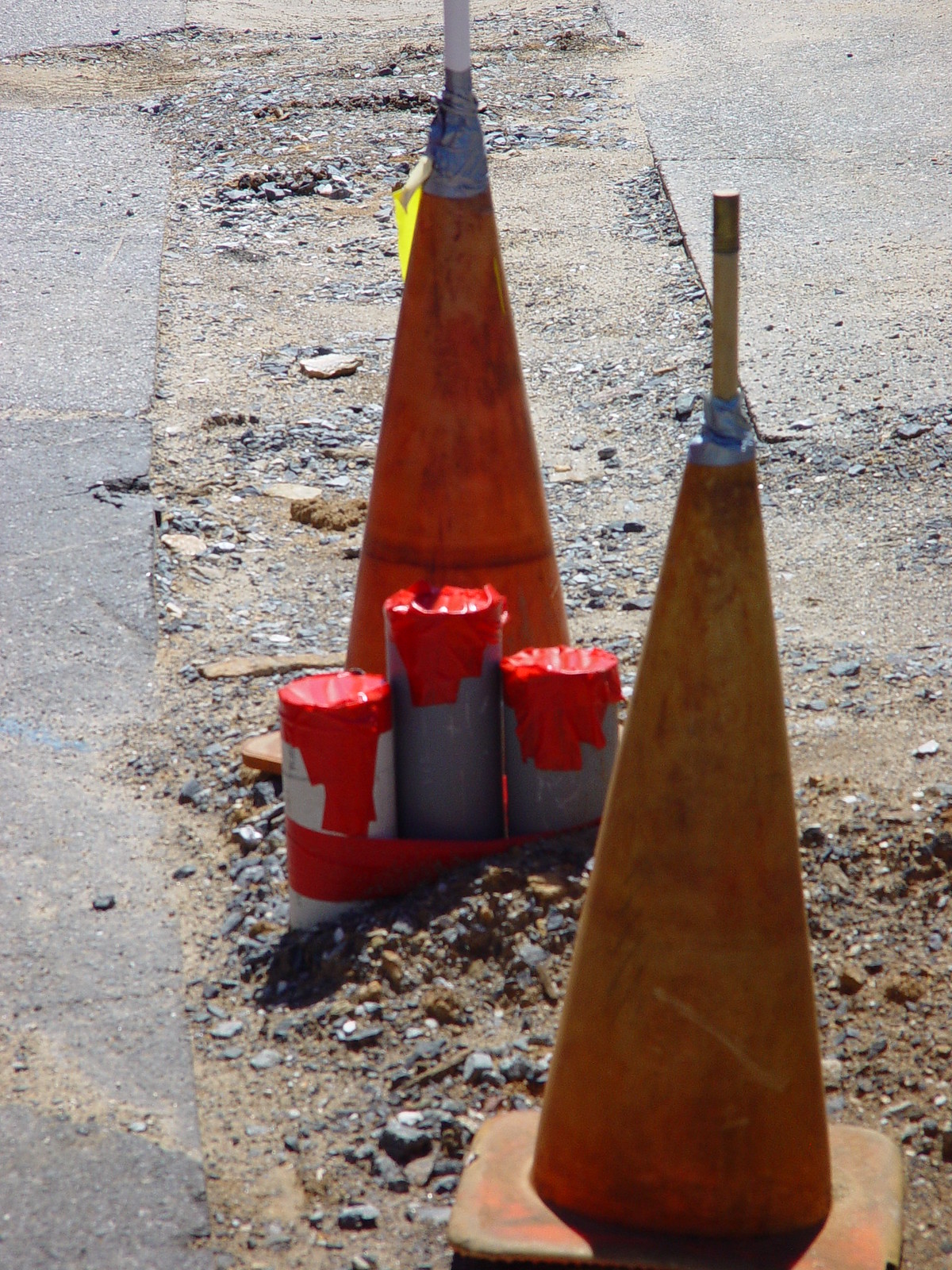This photograph captures a section of a city street undergoing roadwork. The central strip of the image reveals a torn-up portion of pavement, exposing the underlying dirt and scattered with gravel, sand, and small rocks. This strip runs in an L-shape, flanked by old, worn, and chipped pavement with visible potholes on either side. In the foreground, positioned in the lower right corner, is an orange traffic cone with a small length of pipe duct-taped into its upper end. A second cone stands back and to the left of it. Both cones serve to mark the construction zone, warning passersby of the disrupted area. Just ahead, three gray metal pipes protrude from the earth near the rear cone, with red duct tape sealing their tops and securing them together at their base. The scene gives an impression of an area being prepped for extensive road or walkway maintenance.